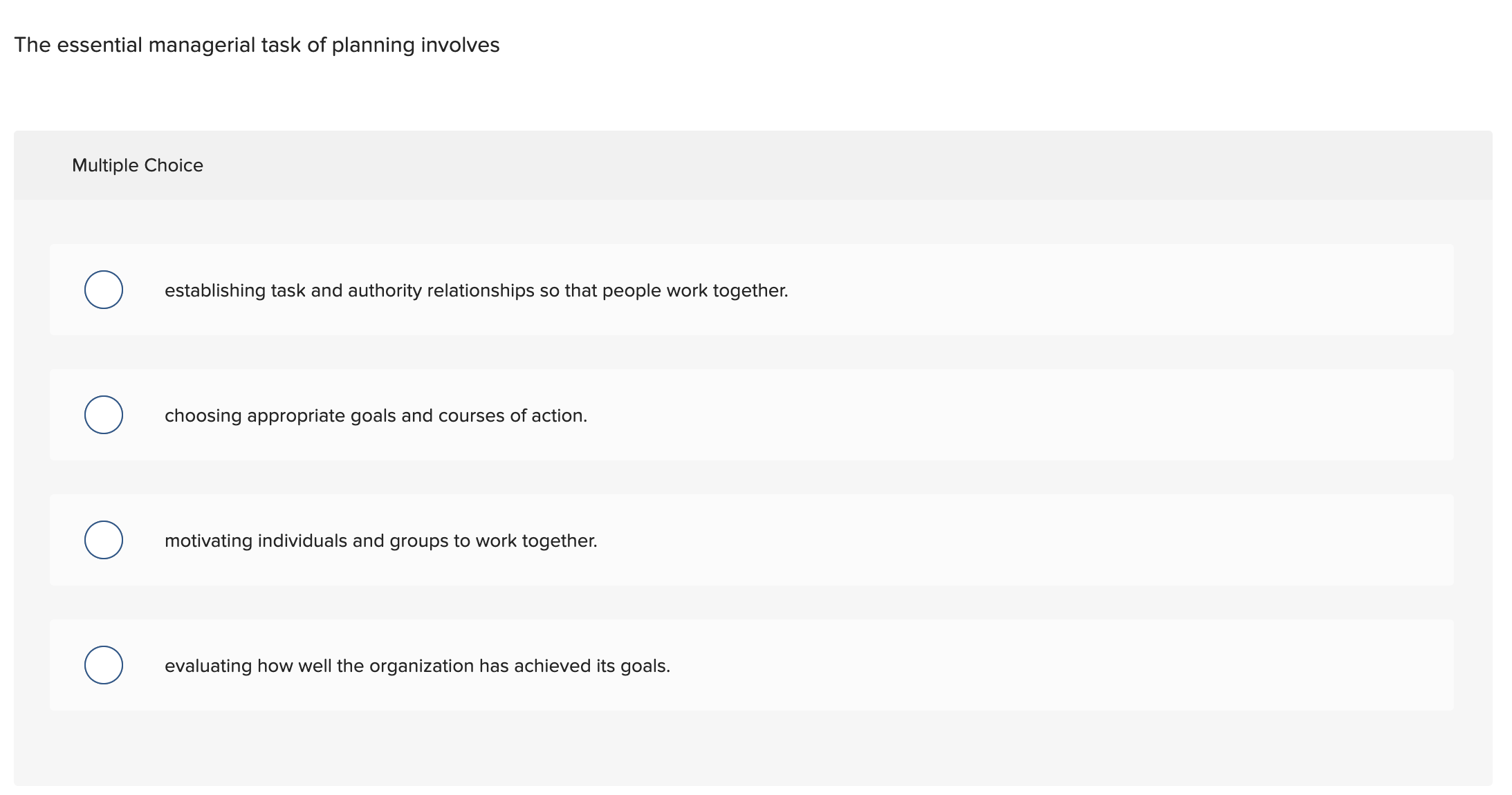In this image set against a stark white background, there is a prominent screenshot featuring a white banner at the top, containing small gray text aligned to the left that reads: "The essential managerial task of planning involves." Below this banner, a light gray box houses four smaller white boxes representing multiple-choice options. At the top of this section is another gray banner that reads: "Multiple Choice." Each of the four options is distinctly listed within these white boxes. The first option reads, "Establishing task and authority relationships so that people work together." The second option states, "Choosing appropriate goals and courses of action." The third option says, "Motivating individuals and groups to work together," followed by the fourth and final option, "Evaluating how well the organization has achieved its goals."